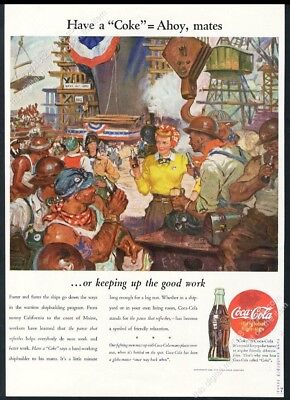This vertically aligned, rectangular Coca-Cola advertisement from the 1950s features a black border and a white background. At the top, it prominently displays the slogan "Have a Coke = Ahoy Mates" in large text. The central image, set against a bar-like backdrop, showcases a lively gathering where men wearing hard hats are enjoying Coca-Cola beverages. Dominantly featured is a woman in the center, dressed in a long-sleeve yellow blouse with a bow tie, a red scarf around her blonde hair, and either brown pants or a skirt. Below the main image, the tagline "...or keeping up the good work" is written. In the lower right corner, there's an illustration of a classic Coca-Cola glass bottle alongside the iconic Coca-Cola logo, a red circle with white script, accompanied by fine print too small to read.